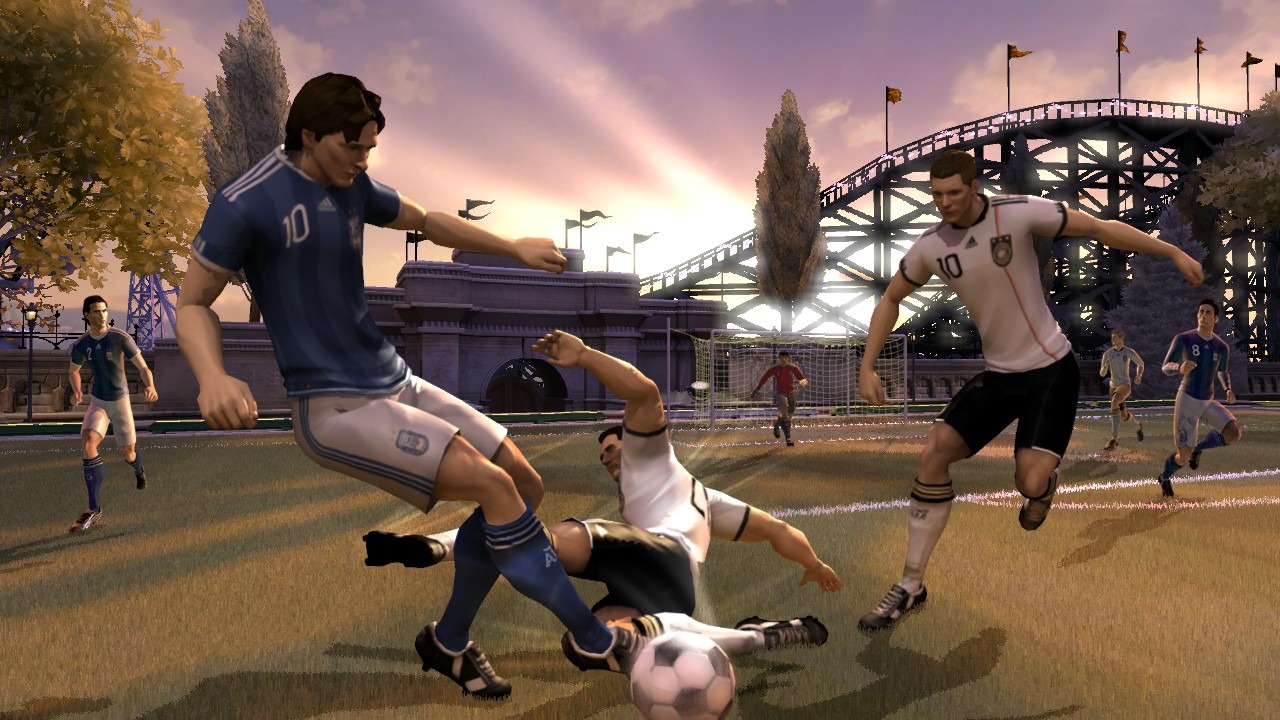In this graphically designed image, reminiscent of a still from a video game, three soccer players converge intensely around a soccer ball. The player on the far left is clad in white shorts and a blue short-sleeved top, his foot poised right next to the ball as he attempts to kick it, arms outspread for balance. Opposite him, another player in a white short-sleeved top and dark shorts rushes towards the ball but remains slightly distanced from the immediate action.

Centrally, a player wearing an identical uniform to the rightmost figure lies sprawled on the ground with his legs outstretched, seemingly in the midst of a slide tackle aimed at intercepting the blue-shirted opponent or gaining control of the ball—or possibly both.

The dynamic scene unfolds on a soccer field bathed in the warm hues of either sunrise or sunset, casting a dramatic light over the action. In the backdrop, several other players are running towards the focal point of the scene, while the surrounding environment is dotted with trees, a building, fluttering flags, and what appears to be a roller coaster, adding depth and context to the intense moment captured.